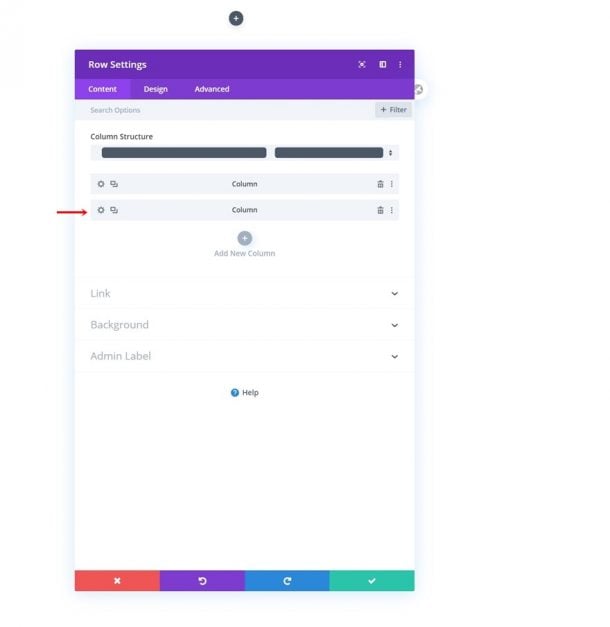The screenshot displays a user interface of a phone application with various design and content settings. At the top, there's a prominent purple box labeled "Row Settings." Below that, in a lighter shade of purple, tabs labeled "Content," "Design," and "Advanced" are visible, indicating different settings options.

The background is white, featuring a section titled "Search Options" on the left and a "Plus Filter" button on the right. Further down, there's a "Column Structure" section, showcasing choices for column layouts. The second column layout option is selected, and a trash can icon is positioned to the right of this option for deletion.

Below the column structure settings, a gray "Add New Column" prompt accompanied by a plus sign is visible. There are several expandable links for further settings: "Link," "Background," and "Admin Label," each with a downward-pointing arrow icon. A small blue circle with a question mark labeled "Help" is also present.

At the very bottom of the interface, there are four colored action buttons: a red box with an X, a purple box with a refresh icon pointing left, a teal box with a refresh icon pointing right, and a green box featuring a checkmark, providing various action options for the users.